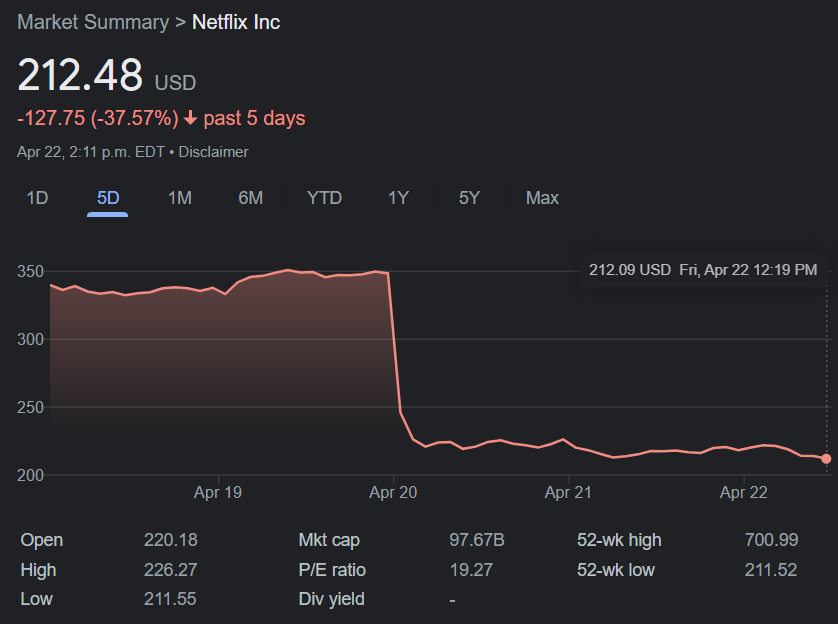This image is a detailed screenshot illustrating the stock performance of Netflix Inc., formatted in a landscape orientation. At the uppermost section, the heading "Market Summary" is prominently displayed, followed by the company name "Netflix Inc." in white text. The current stock price is listed as $212.48, indicating a significant decrease of $127.75, or -37.57%, over the past five days. The data is timestamped for April 22nd at 2 p.m. EDT.

Adjacent to these details is a disclaimer specifying that a five-day chart is being displayed. The chart allows for alternative timeframes including one day, five days, one month, six months, year-to-date, one year, five years, and max. Within the five-day chart, a notable stock drop is observed beginning on April 20th, which continues over the subsequent two days. Additional information highlights that the stock price was $212.09 on Friday, April 22nd at 12.19 p.m.

Further stock details below the chart reveal that the opening price was $220.18, with a high of $226.27 and a low of $211.55. The market capitalization stands at $97.67 billion, and the price-to-earnings (PE) ratio is 19.27.